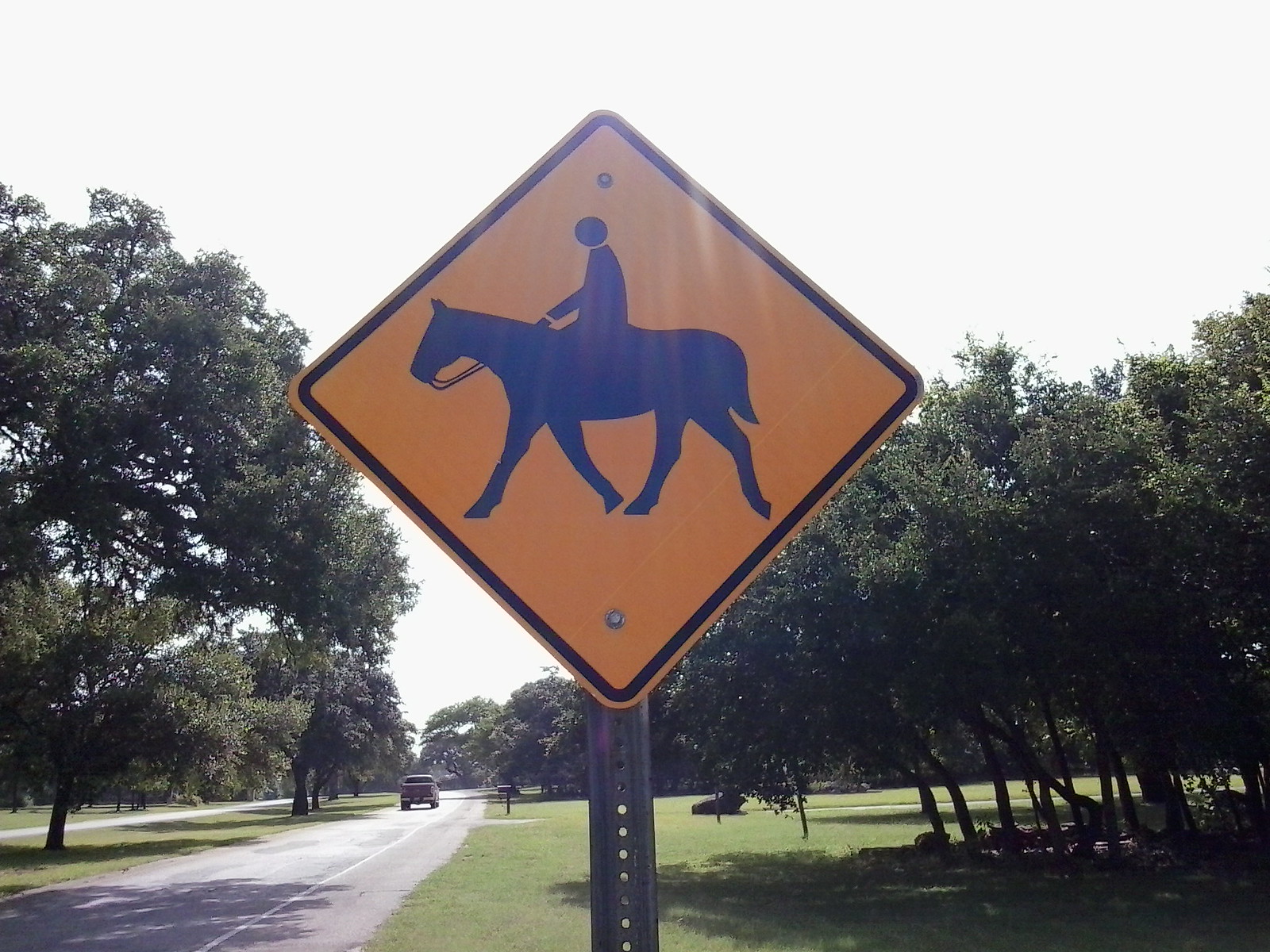The photograph presents a picturesque rural scene with a prominent focus on a cautionary street sign. The diamond-shaped sign, bordered in black with a vibrant yellow background, features a black silhouette of a person riding a horse, signaling a potential equestrian crossing. The sign is affixed to a perforated metallic post using bolts at both the top and bottom.

In the background, the serene countryside unfolds with lush green grass stretching into the distance. A cluster of trees occupies the right side of the image, casting ample shade over the surrounding area. On the left, a narrow road edged with a white line lacks a sidewalk, its asphalt seamlessly blending into the grass verge.

Further up the road, a dark-colored truck is visible, adding a touch of life to the tranquil scene. A grassy median runs parallel to the road, separating it from an adjacent route. This divider, adorned with trees, creates a natural boundary.

In the far distance, the landscape is dominated by towering treetops, their dense foliage a vibrant green. The sky above is a light gray, suggesting an overcast day, yet the daylight indicates that it's taken during daytime hours, evoking a calm and serene atmosphere.